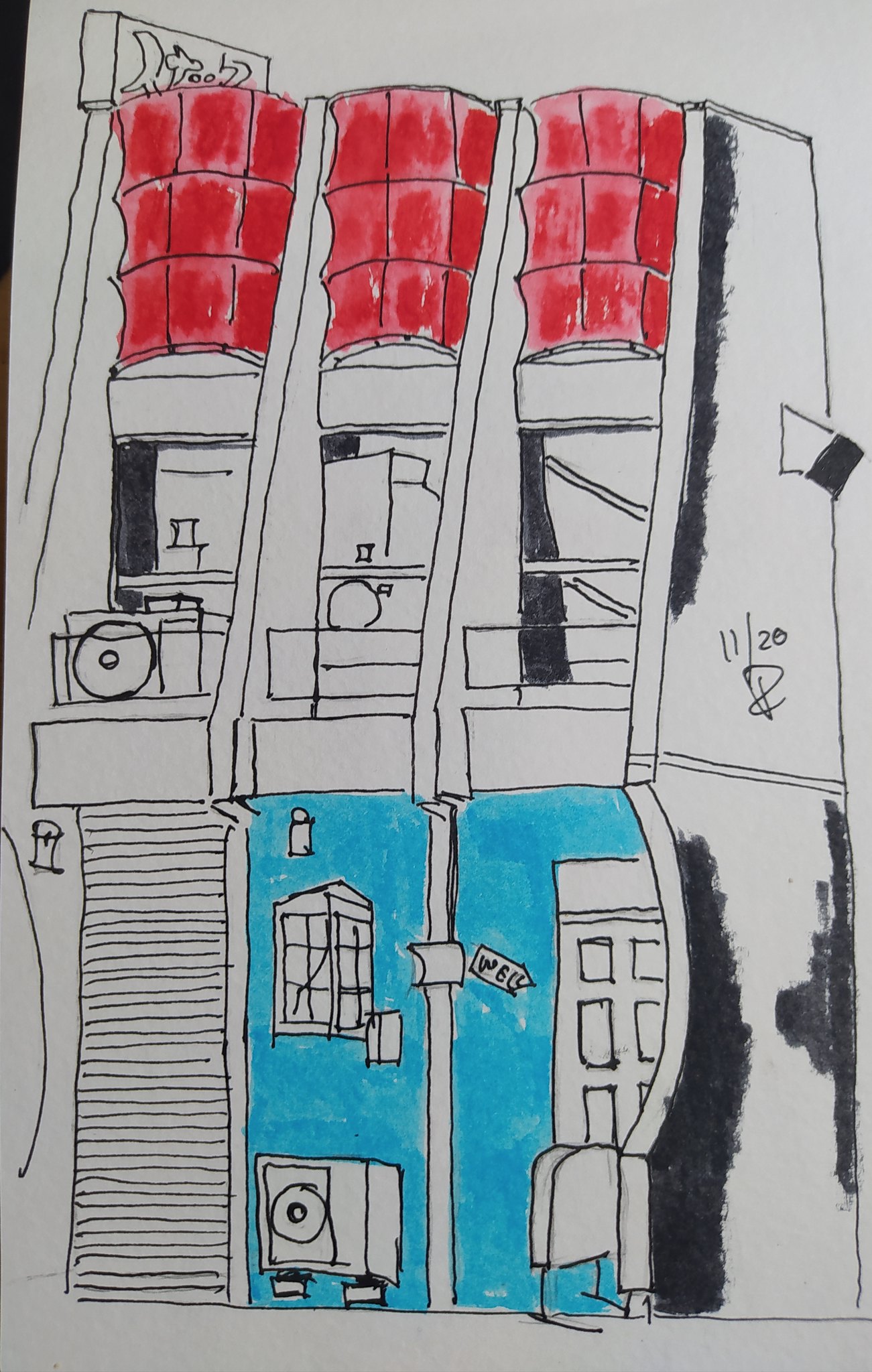This image depicts a detailed sketch of a house or structure, illustrated predominantly with black and white lines, and highlighted with touches of red and blue colored markers. The structure features a roof adorned with three barrel-shaped tubes rendered in red. Above the roof is a black and white sign marked with unrecognizable lettering.

Directly beneath the roof, the design includes various black and white line drawings that likely represent pillars. The right side of the building bears the date "11/20," accompanied by initials that are difficult to decipher. On this same side, the front wall showcases a splash of blue.

There is an intricately drawn window and door on this front wall, and a section of a partially shaded area adjacent to the door. To the left of the door, a line drawing depicts a possible stairway, illustrated with lines within a long rectangle, seemingly extending from the ground level up to the second floor of the building.